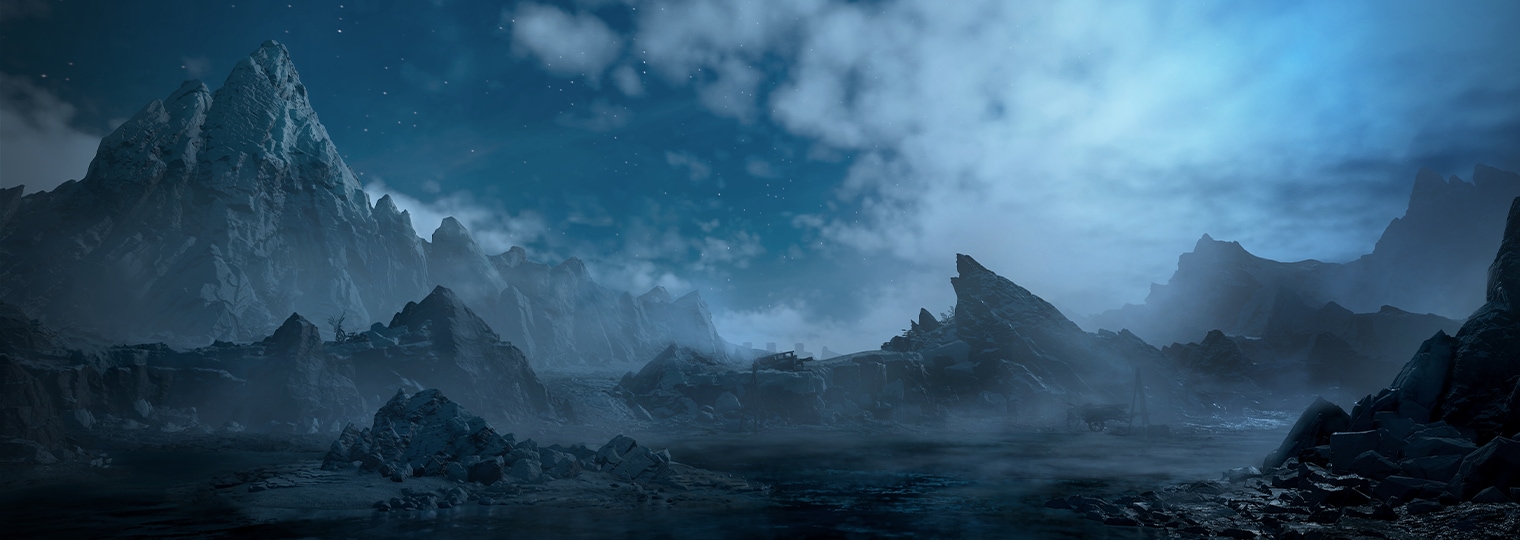The rectangular image vividly captures a surreal and dramatic night setting with a wide landscape of mountaintops. Dominated by hues of dark blue, black, and gray, the picture features a series of jagged mountain ranges that transition from an intense black in the foreground to lighter grays as they recede into the background. The sky above is a dark gray, densely packed with white clouds, especially concentrated on the right-hand side, which are illuminated by what appears to be moonlight. The moon, partly obscured by clouds, casts a ghostly light over the rugged landscape, enhancing the eerie atmosphere. Below, rocky protrusions are scattered around the bases of the mountains, adding to the harsh and raw aesthetic. The leftmost mountain has a tip tinged with a light gray, contrasting with the predominantly dark tones that blanket the rest of the scene. Fog envelops the lower elevations and mingles with the thick clouds above, further intensifying the enigmatic ambiance of this striking nightscape.